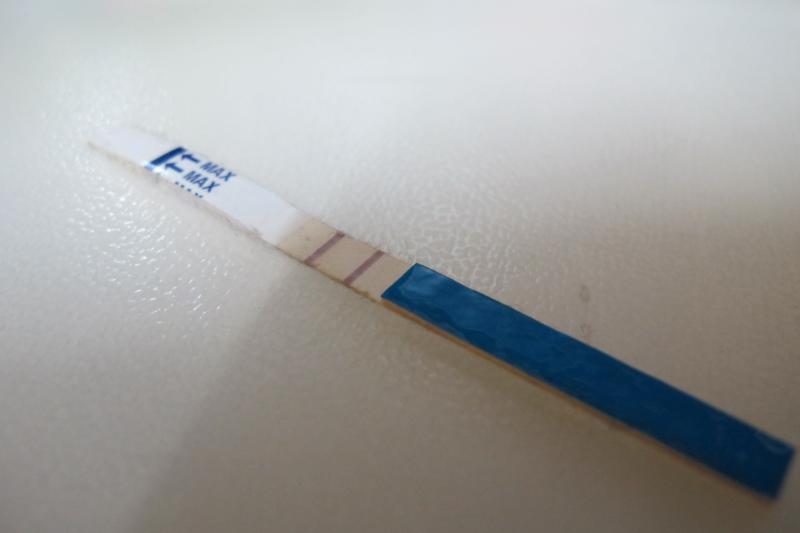The image features a horizontally oriented photograph capturing a test strip used for diagnostic purposes. The test strip spans diagonally from the upper left to the lower right corner, resting on a dimpled white surface. On the right-hand side of the strip, occupying approximately half its length, is a blue area. The left end of the test strip is marked by a blue line labeled "MAX," with accompanying blue arrows indicating the upper limit for the material to be tested. In the center portion of the test strip, there are two parallel purple lines aligned with the MAX mark, serving as indicators for the test results.